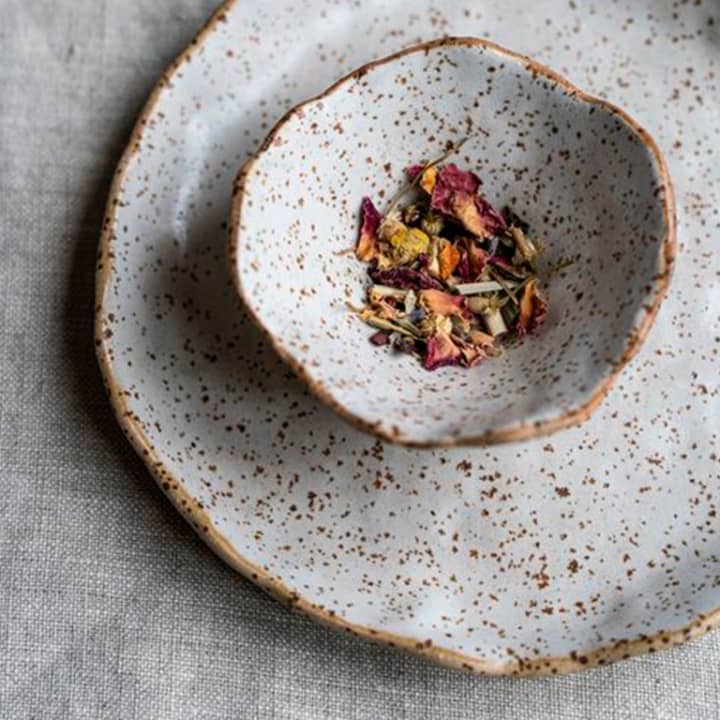The photograph is a full-color, vertically rectangular image captured indoors for artistic purposes. Taken from above, it showcases a pristine white tablecloth serving as a backdrop for a white plate and bowl ensemble. Both the plate and bowl feature an off-white color with brown speckles and a tan rim, giving them a rustic, possibly homemade appearance, emphasized by their slightly irregular edges. The bowl, nested in the middle of the plate, contains a mixture of dried flowers and potpourri leaves in shades of red, orange, and green, along with small sticks, adding a textured, aromatic element to the composition. The overall image is cropped, cutting off parts of the plate at the top and on the right, yet it beautifully captures the artistic and visually interesting display of the china and its natural contents.